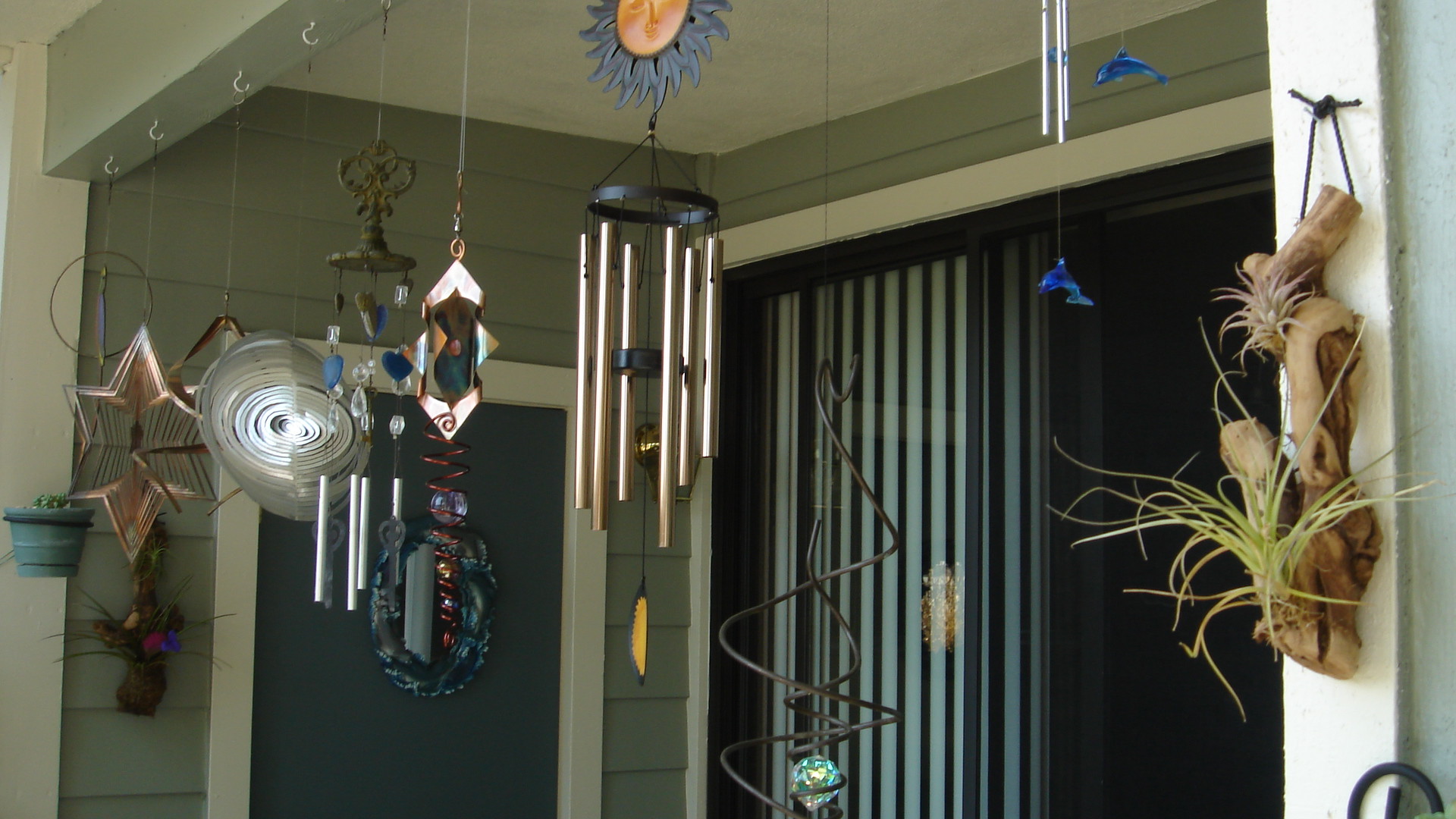The image depicts a porch or deck, likely in an apartment complex, adorned with a variety of wind chimes and decorations. Hanging from the ceiling are about nine to ten wind chimes of different shapes and sizes, including traditional ones with long bars, a spiral-shaped one, and a star design. One prominent wind chime features an orange sun with black rays. Other decorations include a golden star, a dark brown piece of wood with a black string and a green plant attached, and various items with black and yellow color schemes. The setting also includes sliding glass doors with shades, and elements like a white pillar, a mesh wire at the bottom, and a black window frame on the right side. A green pot plant adds a natural touch to the predominantly decorated space.